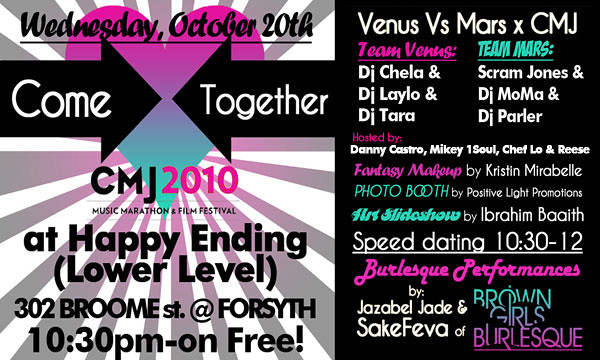This vibrant event flyer for the CMJ 2010 Music Marathon and Film Festival, scheduled for Wednesday, October 20th at Happy Ending, Lower Level, 302 Broome Street at Forsyth, kicks off at 10:30 PM and promises a fun night on the house. The left side of the flyer features a retro sunburst pattern in white, gray, and pink with a central pink, blue, and green heart. Black arrows point inward toward the heart with the text "Come Together" in white. Above the heart in black font are event details. 

The right side of the flyer, striking with its black background contrasted by vibrant pink, green, and beige elements, announces the "Venus vs. Mars X CMJ" showdown. Team Venus, featuring DJs Chela, Lalo, and Tara, stands in friendly competition against Team Mars, comprising DJs Scram Jones, MoMa, and Parlor. The event is hosted by Danny Castro, Mickey One Soul, Shefflo, and Reese.

Additional attractions include Fantasy Makeup by Kristen Mirabel, a Photo Booth by Positive Light Promotions, an Art Slideshow by Ibrahim Baith, Speed Dating from 10:30 to midnight, and exhilarating burlesque performances by Jezebel Jade and Saki Fiva, presented by Brown Girls Burlesque.